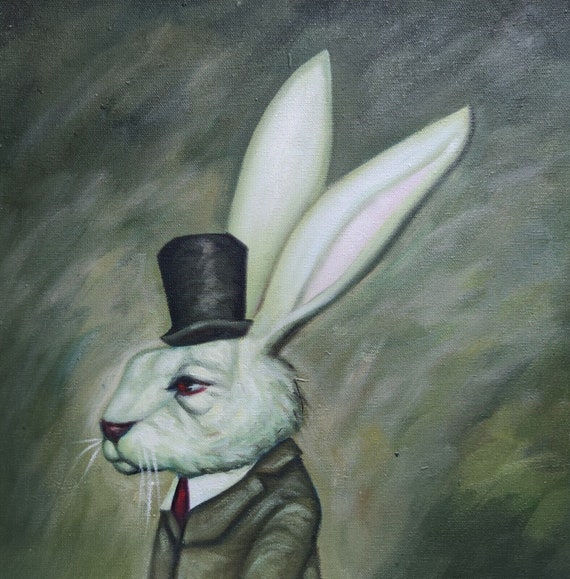This image is a detailed painting depicting a white rabbit dressed in formal attire, positioned towards the bottom left of a square canvas. The rabbit stands upright like a human, wearing a black shiny top hat that adds to its anthropomorphic appearance. It dons a brownish-gray blazer jacket with white accents and a red tie over a white collared shirt. The rabbit, facing towards the left, displays a somber expression with bags under its red eyes, a pinkish-red nose, and white whiskers surrounding its mouth. Its long white ears, which have pink on the inside, extend up and slightly backward, reaching towards the upper right of the image. The background consists of a mix of drab, cloudy colors including shades of gray, white, green, yellow, and black, creating a smudged, abstract backdrop that contrasts with the detailed portrayal of the rabbit.